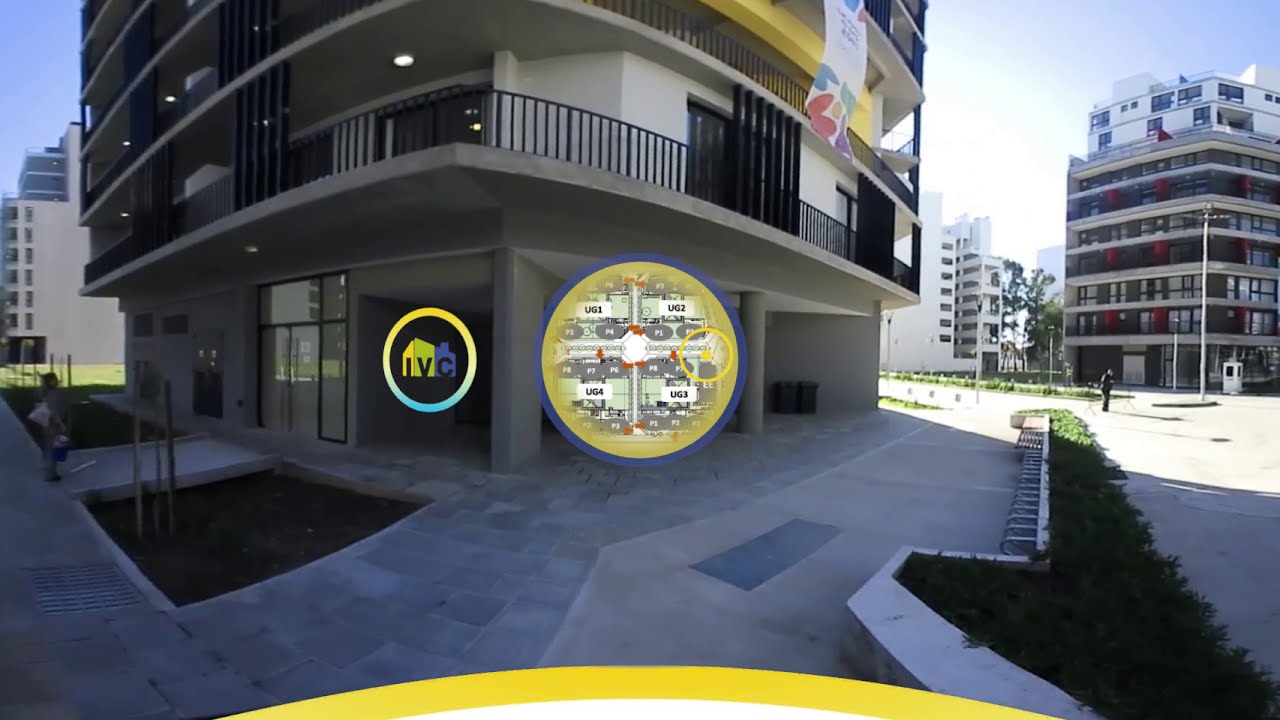The image depicts a bustling urban setting, focusing on a multi-storied, square-shaped apartment building with an off-white facade accented by yellow ledges. Each floor features balcony areas enclosed by railings. A banner adorned with multicolored flowers hangs prominently from the building. The ground below is predominantly concrete, interspersed with tile walkways guiding pedestrians, and features a raised flowerbed with a small amount of greenery. Central to the image, on the lower floor of the building, are two significant circles; one contains a symbol with the letters IBC and an image of a house, while the other circle appears to depict a colorful map with labeled locations. To the left and right of the main building, additional buildings of similar aesthetic stand, enhancing the urban landscape. A person is seen standing near the leftmost building, with another individual in the distance on the right. The scene, captured during daytime, showcases a well-maintained and active city environment with architectural and natural elements blending seamlessly.